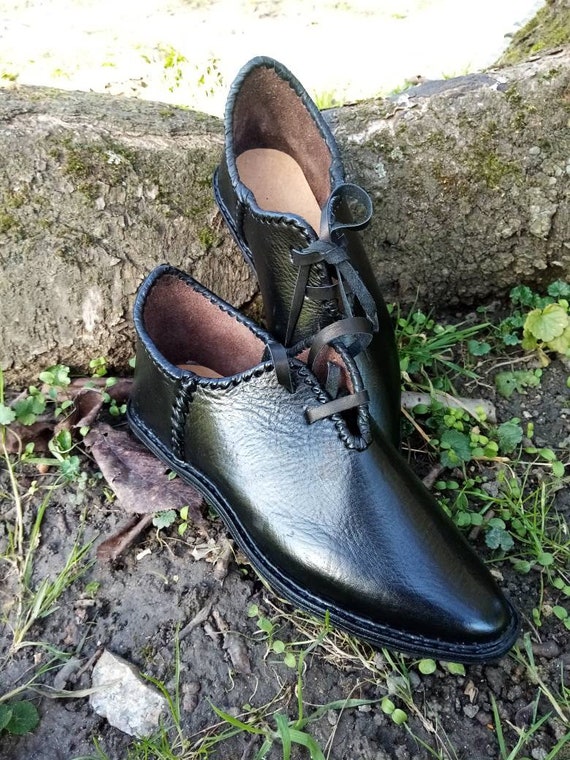The photograph features a stylish pair of men's dress shoes, characterized by their pointed toes and sleek black leather exterior. Each shoe is anchored by a thin black sole. The interior showcases a contrasting brown and tan leather, visible due to their positioning. Foregoing traditional laces, the shoes are secured by a black leather strap threaded through four holes at the front. The front shoe lies flat on a dark brown earthy surface, interspersed with sparse vegetation, such as clover and grass strands. A dead leaf is tucked under its heel, adding a rustic touch. The back shoe is artfully propped up, its heel elevated by a large, gray boulder speckled with moss and other vegetation. The shoes are staged in an outdoor setting, with detailed heavy stitching along the edges and down the sides, giving them a modern yet rustic appeal. The image itself is rectangular, with its length twice that of its height, encapsulating this elegant and natural composition.